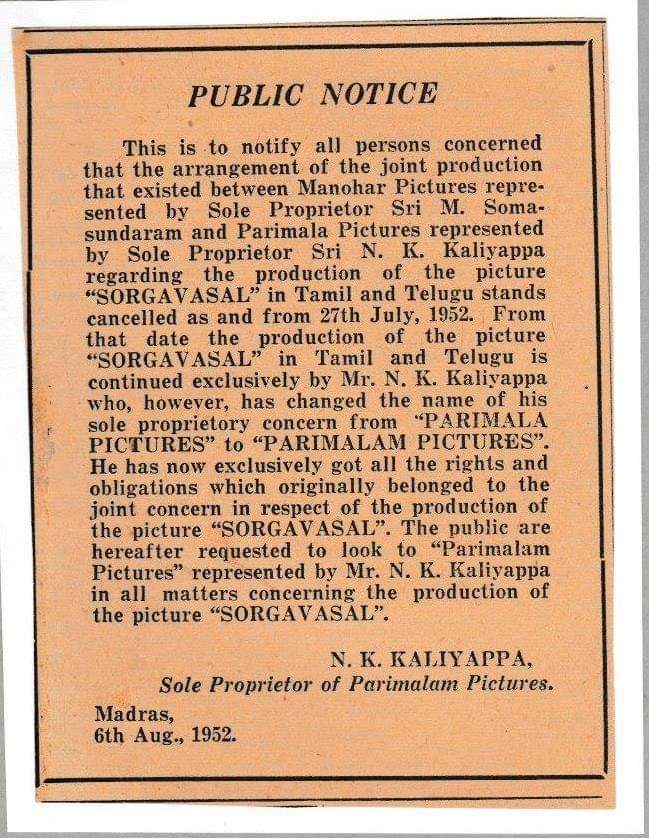The image depicts an old, faded poster with a light brown background and black text, resembling a yellowing newspaper clipping. The rectangular poster is vertically oriented with a thin black border. At the top, in capital letters, is the title "PUBLIC NOTICE". Below the title, the notice reads:

"This is to notify all persons concerned that the arrangement of the joint production that existed between Manohar Pictures, represented by sole proprietor Shri M. Soma Sundaram, and Parimala Pictures, represented by sole proprietor Shri N.K. Kaliyappa, regarding the production of the picture Sorgavasal in Tamil and Telugu stands cancelled as of 27th July 1952. From that date, the production of the picture Sorgavasal in Tamil and Telugu will be continued exclusively by Mr. N.K. Kaliyappa, who has changed the name of his sole proprietary concern from Parimala Pictures to Parimalam Pictures. He now exclusively holds all rights and obligations that originally belonged to the joint concern with respect to the production of the picture Sorgavasal. Henceforth, the public is requested to address all matters concerning the production of the picture Sorgavasal to Parimalam Pictures, represented by Mr. N.K. Kaliyappa."

The notice is signed by N.K. Kaliyappa, Sole Proprietor of Parimalam Pictures, Madras, dated 6th August 1952.